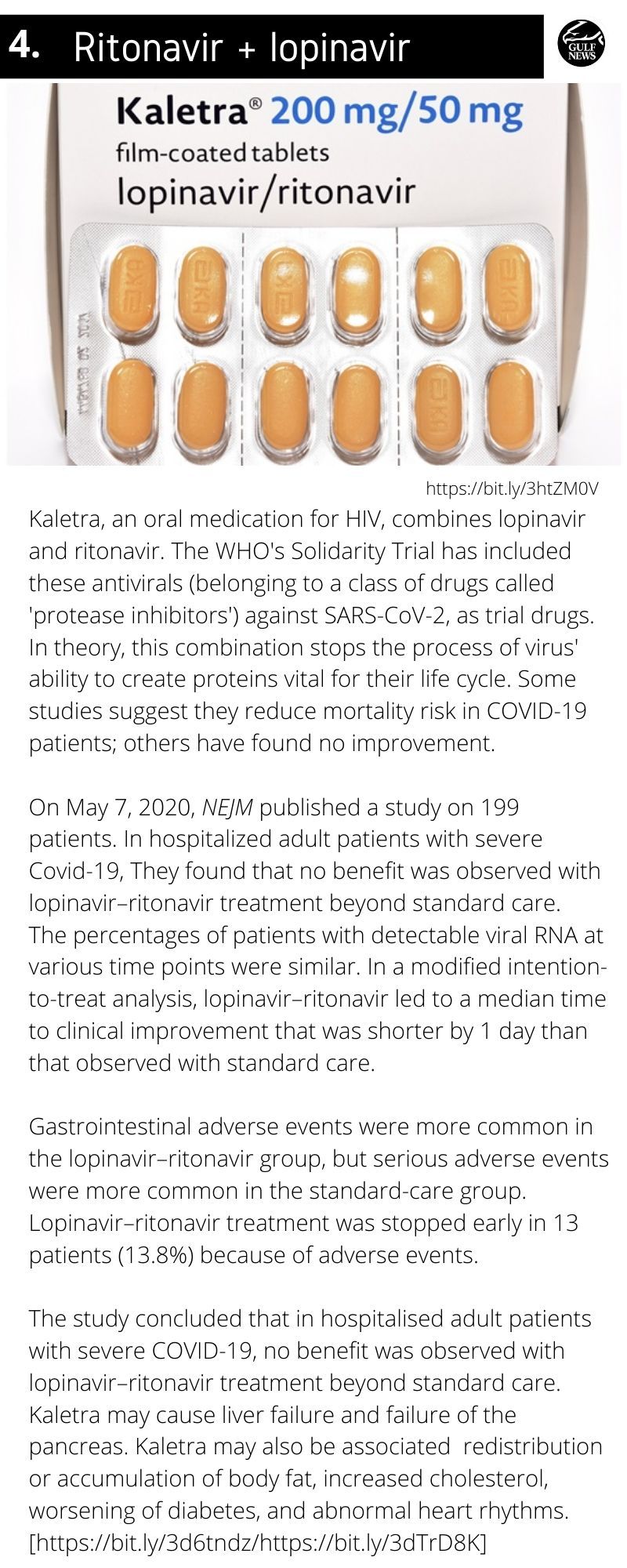This screenshot features detailed information about Coletra 200mg/50mg film-coated tablets, an oral medication used for HIV treatment that combines the antiviral agents lopinavir and ritonavir. Coletra belongs to a class of drugs known as protease inhibitors, which work by inhibiting the virus's ability to produce essential proteins, thus disrupting its life cycle.

In response to the COVID-19 pandemic, Coletra was included in the WHO Solidarity Trial as a potential treatment against SARS-CoV-2. The rationale behind this inclusion is the theoretical capacity of lopinavir and ritonavir to inhibit viral replication. Some initial studies have suggested that these drugs may reduce the risk of mortality in COVID-19 patients; however, the findings have been inconclusive or contradictory.

On May 7, 2020, the New England Journal of Medicine (NEJM) published a significant study involving 199 hospitalized adult patients with severe COVID-19. This study concluded that the lopinavir/ritonavir combination did not provide additional benefits over standard care. The outcomes showed no significant difference in the percentages of patients with detectable viral RNA at multiple time points. Consequently, any modified intention-to-treat analysis echoed these findings, indicating that Coletra did not improve clinical outcomes in the treatment of severe COVID-19 beyond what standard care offers.